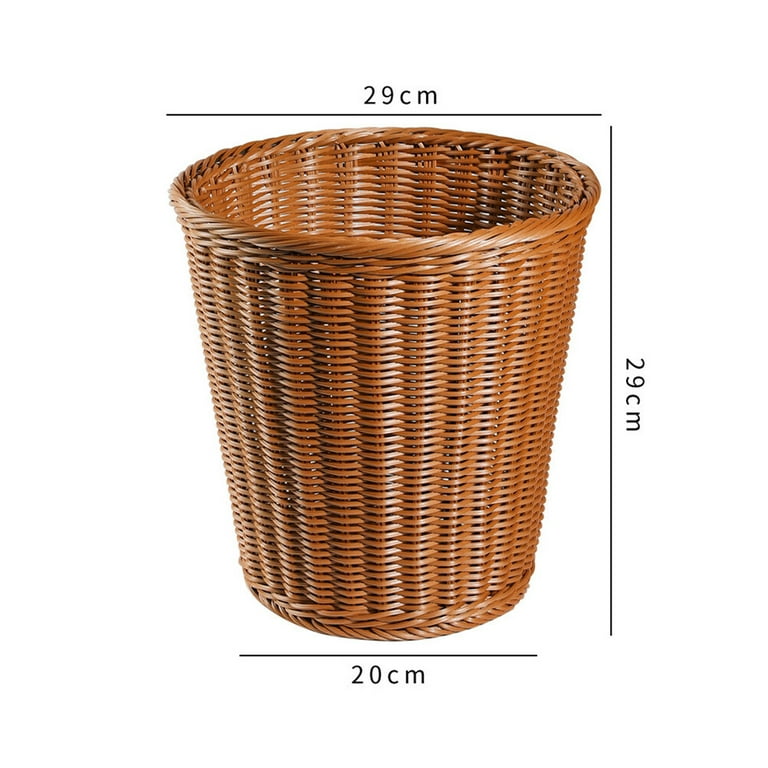This image is a color photograph of a brown woven wicker basket, isolated against a plain white background. The basket, constructed from light to medium brown organic materials, features horizontal weaving with vertical ribbing. It has a round cylindrical shape that tapers wider at the top and narrows towards the base. The basket's dimensions are clearly marked with black diagram lines: a horizontal line at the top shows the basket's opening at 29 centimeters, a vertical line on the right side matches the basket's height at 29 centimeters, and another horizontal line at the bottom indicates the base width of 20 centimeters. The basket's tightly woven structure suggests it could be used for various purposes such as a trash can with a liner, a plant holder with an inner lining, or simply as a decorative object. Despite its relatively small size, it could also potentially hold lightweight items like blankets.